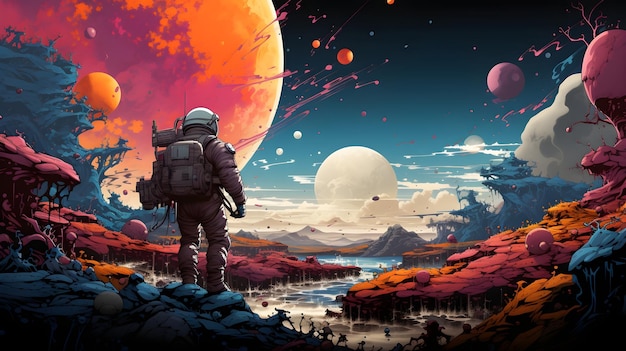An animated digital artwork features an astronaut in a dark brown spacesuit with a white helmet, backpack, antennas, and a pack on his left side. He stands on a rugged, alien terrain adorned with prominent tree roots and mountains in hues of blue, red, and orange. In front of him, a river meanders from the center of the image towards the bottom, transforming from blue to silver. The sky above is a striking blend of blue and black with surreal, blood-like splotches floating in the air.

The backdrop includes two imposing mountains capped with ethereal clouds. To the upper left, a giant orange planet fades into purplish and pink hues, stretching nearly to the center of the image. Adjacent to it is a fairly large white planet. A smaller purple planet sits in the upper right corner. Some additional smaller planets and mysterious paint-like drops are scattered across the sky, adding to the otherworldly atmosphere. The astronaut stands on the center-left, gazing toward this alien landscape, a city hinted at in the middle distance.